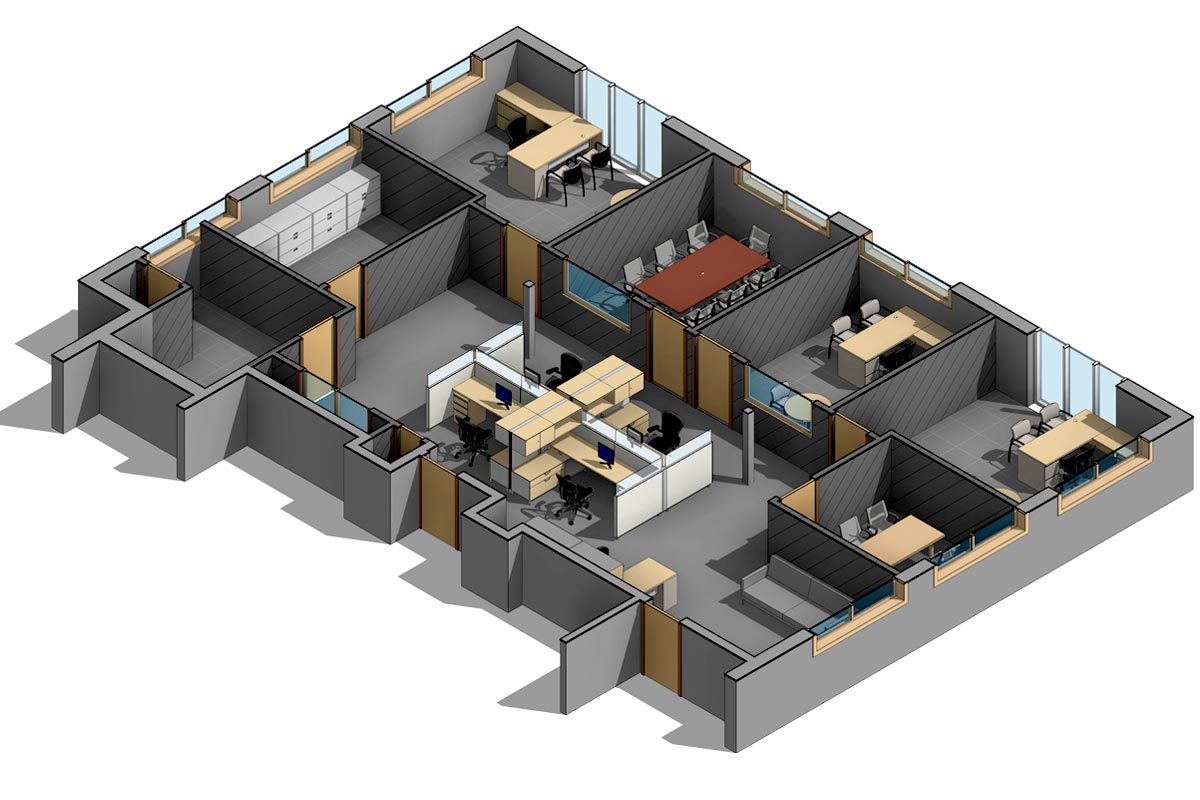The image is a detailed, computer-rendered, three-dimensional illustration of one floor of an office building, viewed from a three-quarter perspective with the roof removed to reveal the interior layout. The walls, carpets, and boundaries are all shades of gray, creating a cohesive look throughout. Central to the image is an open area with four cubicles arranged in a more open workspace setup. Surrounding this central space are several individual offices, each furnished with similar desks and chairs. Notably, the topmost office features an L-shaped desk, while another office below it contains a red desk and multiple chairs, identifying it as the meeting or conference room with a long brown table and seven chairs. Additionally, if you enter through one of the front doors and make a left, there is a room dedicated to storage, filled with filing cabinets. The building's layout also includes various doors leading to small windows and larger floor-to-ceiling windows, enhancing the open feel of the space.